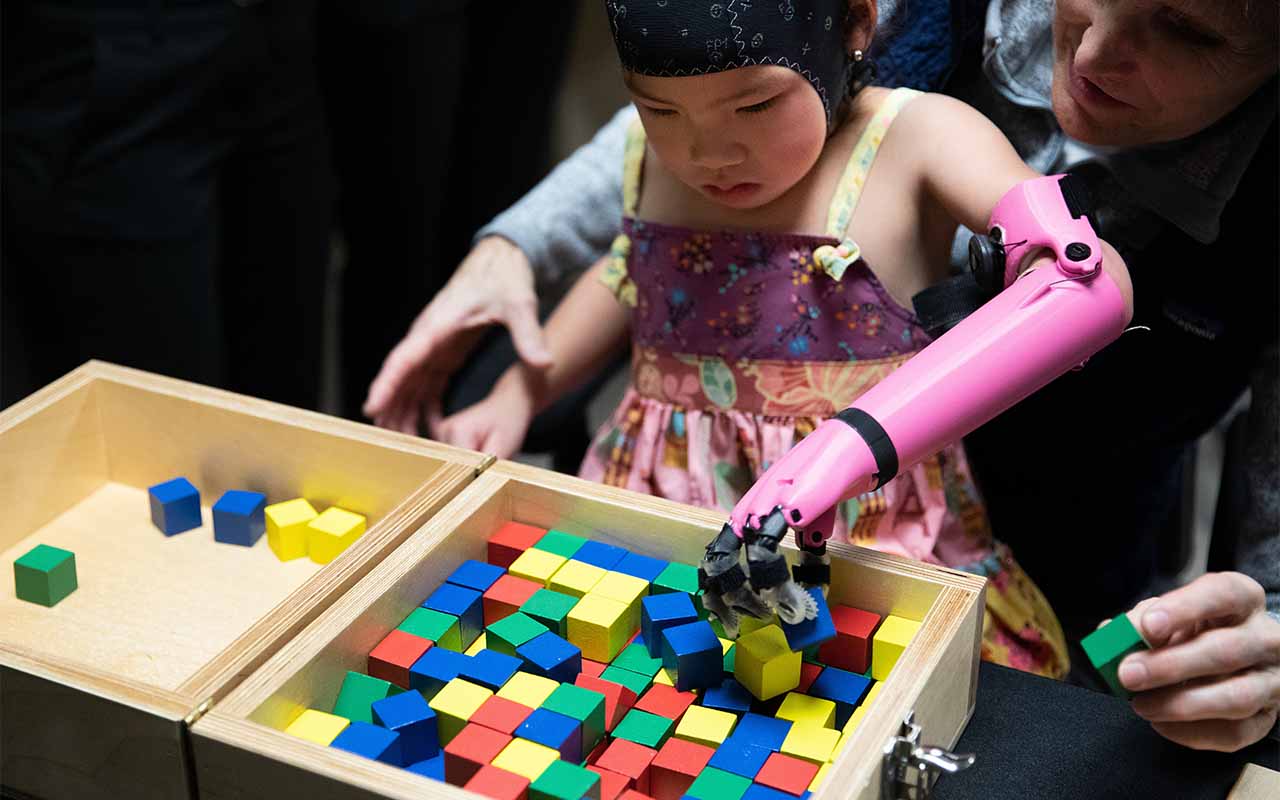In this square indoor photograph, the focal point is a young Asian girl wearing a black and white hood that covers her hair and chin. She is dressed in a multicolored spaghetti-strap dress that features purple, yellow, peach, and pink hues. The girl's left arm is an advanced pink prosthetic device with black fingers that have white, rubber-textured tips. She is concentrating on picking up and manipulating multicolored blocks that are nestled within a large wooden box, positioned in the lower left of the image. The box contains numerous blocks in shades of blue, green, red, and yellow, while its open lid only holds two yellow, two blue, and one green block. To her right side, the protective presence of an adult is visible, with their arms gently wrapped around her. The adult, who may be male or female, holds a green block and appears to be either steadying or reassuring the child as she practices using her prosthetic arm to grasp the blocks. Both the girl and the adult sit on a darkened background, bringing full attention to their learning and bonding moment.